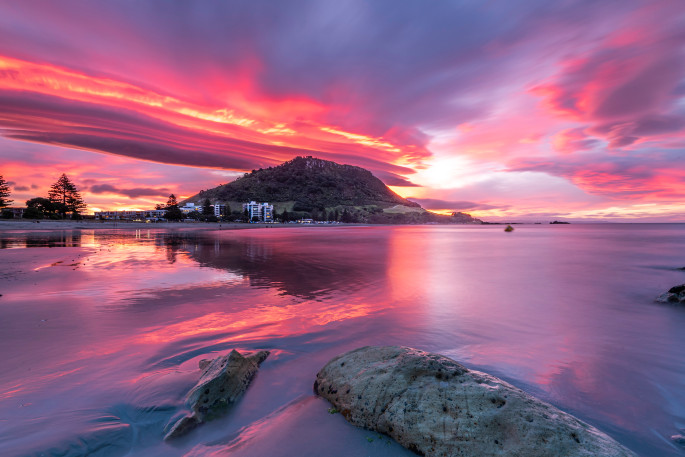This landscape image captures a picturesque outdoor scene featuring a serene water body that occupies the bottom half of the picture. Scattered grey rocks line the foreground, while the water itself, imbued with the soft pinks, yellows, and purples of the reflected sky, glistens in the light of either a setting or rising sun. The central focal point of the image is a small, island-like mound, potentially green or brown, with the tiny white speckles of buildings or hotels dotting its side. To the middle left, the silhouette of a tree adds to the natural beauty. The top half of the photograph is dominated by a breathtaking multicolored sky, showcasing a blend of blues, yellows, reds, and oranges. Wispy, multicolored clouds contribute to the ethereal atmosphere, further enhanced by a purple haze. The result is a harmonious blend of land, water, and sky that creates a tranquil and captivating scene.